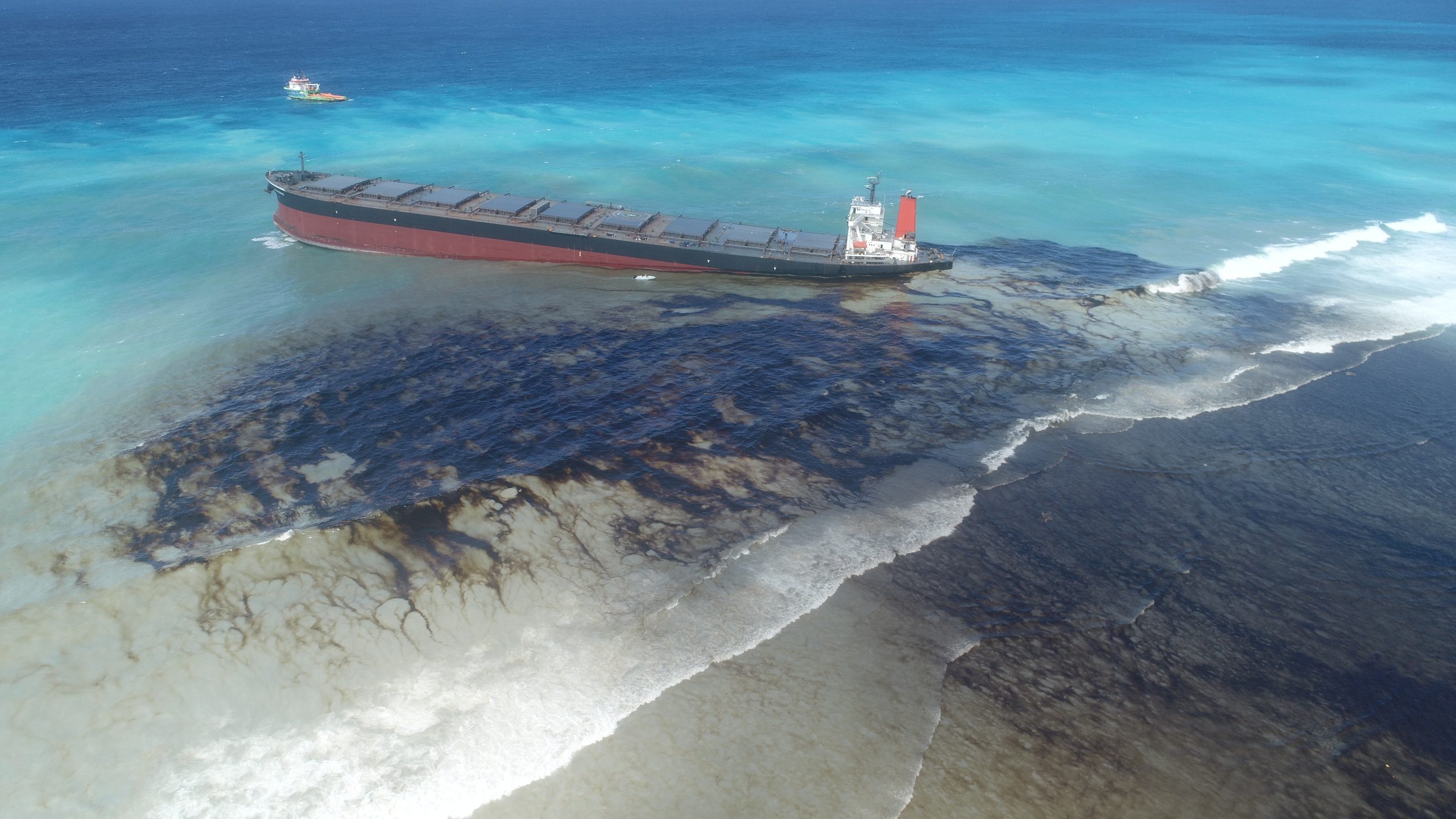The image depicts an actual photograph featuring a large cargo ship or barge, possibly an oil tanker, that appears to be stranded close to a shore. The ship has a stark color contrast, with a black upper section and a dark copper-red lower hull. It is equipped with a white cabin and an orangey flag or chimney structure. The front of the ship is visibly sunken, with more of the vessel elevated at the back, indicating part of it is submerged.

The scene shows clear, beautifully varying water, ranging from light blue to darker blue shades as it stretches into the distance. Notably, a significant oil spill is evident, with a substantial, dark, oily mass contaminating the water around the ship and reaching the shore, creating an unsightly and dangerous situation. The spill is especially prominent on the right side of the image, where the black residue has already tainted the beach.

In the distance, a small tugboat can be seen on the top left, likely assessing the situation or attempting to assist. Additionally, on the stern of the grounded ship, there is a person dressed in an orange raincoat, standing and seemingly awaiting help. The overall image captures a dramatic and distressing maritime accident, underscored by the environmental impact of the evident oil spill.